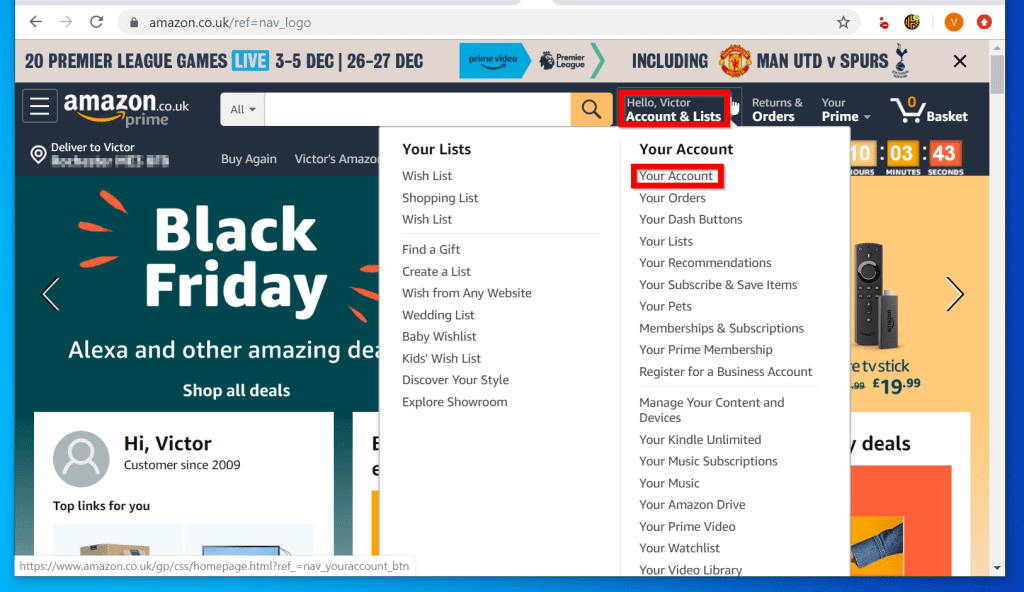This is a detailed caption for the described image:

---

Screenshot of the Amazon.co.uk homepage, displaying the URL "Amazon.co.uk/ref=nav_logo" in the address bar. The page features a gray header at the top with text promoting "20 Premier League games live, 3-5 DEC, 26-27 DEC" and a blue Prime Video icon next to the text "including Man UTD v Spurs." Below the header is a search bar, and to the right of the search bar, the text reads "Hello, Victor Accounts & Lists," which is highlighted by a red rectangular box. A dropped-down white box appears below "Accounts & Lists," containing the menu items, with another smaller red rectangular box highlighting "Your Account" at the top right of the dropdown. Other items listed in the dropdown box include "Your Orders," "Your Dash Buttons," "Your Lists," and "Your Recommendations."

---